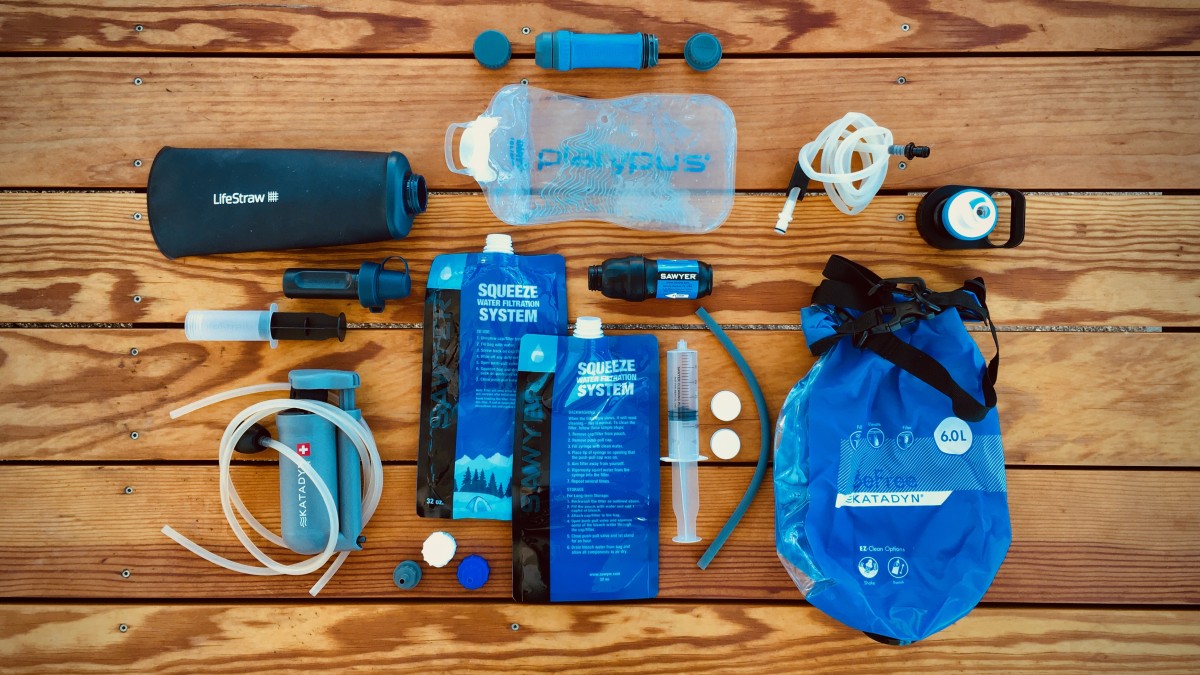The image portrays a detailed layout of a portable hydration system spread across a lightly stained, wooden table, with visible wood grains. Central to the display are multiple components used for filtering and carrying potable water, predominantly in blue with some white and black items. Key items include a dark blue water bottle branded "Life Straw", hinting at the manufacturer. Another clear bottle of similar shape and size is present. Two squeezable bags labeled "Squeeze System" and branded "Sawyer" are designed for water filtration, though the accompanying instructions are not legible. 

A noticeable part of the setup is a blue flexible bag inscribed "Be Free Kataydin," capable of holding six liters, alongside a smaller object appearing like a water pump paired with Nalgene tubing, marked with the Kataydin brand and its Swiss cross logo. The array also includes several tube-like parts, intertwined white tubing, syringes seemingly for pushing water through filter discs, various caps, and small cylinder-shaped devices. At the top of the layout, three small blue objects and a black object add to the intricate assortment of approximately 15 to 20 pieces, suggesting multiple ways to obtain and filter fresh water while hiking or in other outdoor activities.